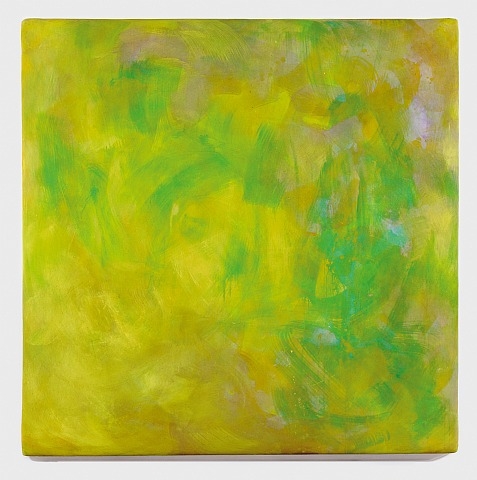This image features a square, abstract painting on a canvas with a solid light gray background that slightly extends beyond the painting. The artwork is predominantly characterized by vibrant yellow brush strokes, particularly dense on the left side, creating a vivid and intense visual experience. Green brush strokes weave diagonally from the top left to the bottom right, with a concentration of green on the bottom right. Brown strokes subtly augment the composition around the top edges, while sparse white or light gray strokes can also be observed, blending into the canvas in sections. The painting has a spontaneous, unfinished appearance, with thick strokes going in various directions and some gaps revealing the white or light gray canvas underneath. Despite the seemingly random application of colors, the arrangement of yellow, green, brown, and white gives the piece a dynamic and captivating essence.